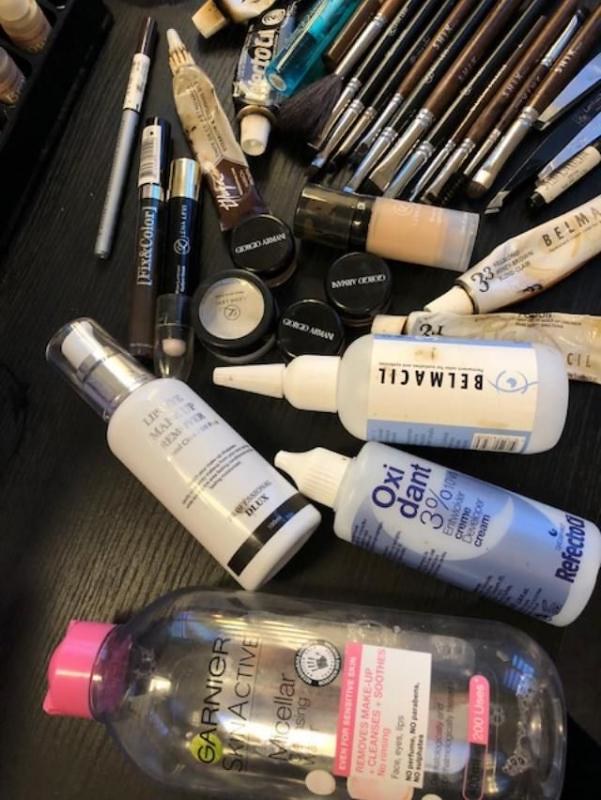In this detailed vertical photograph, a diverse assortment of makeup and personal care products is artfully arranged on a dark brown, horizontally-etched surface. The photo is thoughtfully composed, capturing a variety of items in organized disarray.

At the top edge of the photograph, particularly toward the center and right, a collection of makeup brushes is prominently featured. The handles of these brushes extend off the top right edge, while their bristle heads point diagonally toward the center, aiming towards the lower left corner. These brushes vary in size, showcasing both large brush heads and smaller, more delicate ones, covering approximately the top third of the image.

Adjacent to the brushes, in the top center, resides a small cylindrical tube with a striking turquoise body and black accents. Flanking it, another tube with a blue body adorned in bold white font and capped with white, appears to suggest a squeezable item. A different tube, sporting a dark and light brown body with a white top, is positioned nearby. Its white cap points upward, slightly left of center near the top edge, while the blue tube's white cap points downward.

To the top left of center, a thin stick of eyeliner stands out with a gray base, white label, and brown top, angled towards the upper left portion of the photograph.

Centrally located within the image are four small circular containers. Three are topped with black lids bearing white fonts, while the fourth features a clear center encircled with black, revealing its contents.

Nestled beside these containers are additional makeup pieces. A notably black item with a clear, white-tipped point and a silver back lies left of center, directed downward. Another brownish makeup pencil, labeled at the top, points upward.

Further down, near the center right, a frosted clear foundation bottle filled with light brown or tan makeup and sealed with a black cap, stands out. Its orientation is slightly tilted, with its top pointing to the upper left.

Continuing along the middle right side, several makeup tubes, primarily white, peep in from the edge, their caps directed towards the middle of the frame. Tucked into this array are four bottles, all facing left. Three bottles are white, with two adorned in black font and the third, touching the right edge, highlighted by blue font. Completing this assembly is a clear bottle at the bottom edge, partially obscured, distinguished by its pink plastic cap.

The strategic arrangement and variety of textures and colors provide a rich narrative of beauty essentials, inviting the viewer to explore each meticulously-placed item.